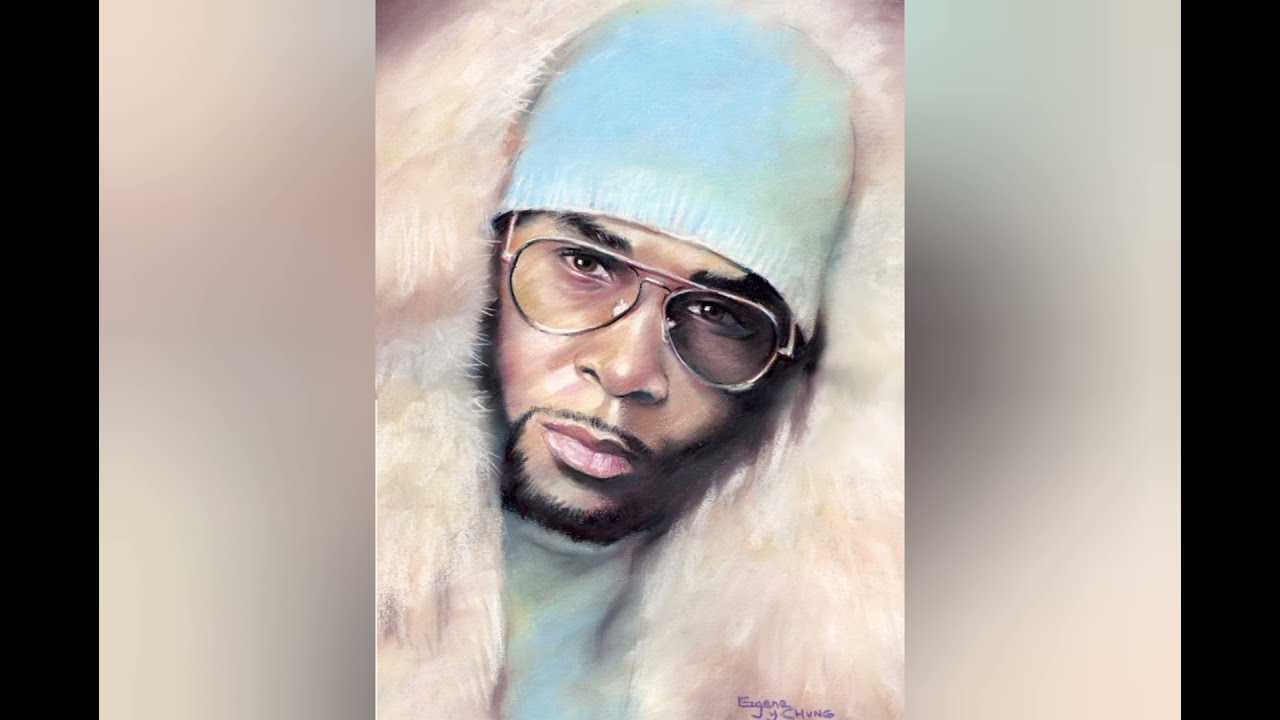This highly realistic and colorful painting portrays an African-American man, who bears a resemblance to Rhythm and Blues singer R. Kelly. The artwork captures his distinct features, including dark skin and a sophisticated beard and handlebar mustache combination. His head is adorned with a light blue beanie that matches the top portion of his shirt, which peeks out from beneath a cream-colored fur shawl enveloping his head and shoulders. He wears remarkably clear aviator glasses through which his eyes are fully visible. The absence of discernible lines and a soft smudge painting technique give the image a polished and photo-like quality, adding to its lifelike appearance. This meticulous piece is signed at the bottom by the artist, Eugene Y. Chung.